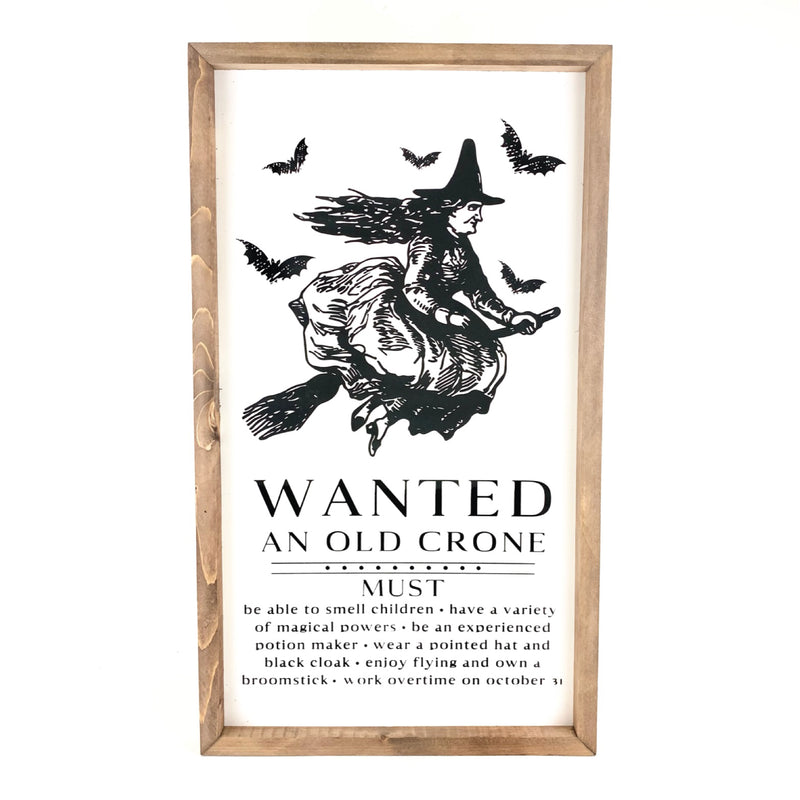The image depicts a vertically aligned rectangular sign with a medium brown wooden frame, showcasing visible wood grain and knots, particularly on the left side. Set against a white background, the black and white illustration within the frame features a witch in a full-length dress, flying rightward on a broomstick with her hair streaming several feet behind her, and wearing the classic pointed hat. She is surrounded by five bats, two in front, one above her head, and two behind. The witch's facial expression appears mean. Below the witch, large, bold, black capital letters headline the sign with "WANTED," followed by "AN OLD CRONE." Beneath this headline, text in all caps elaborates on the witch's qualifications: "MUST BE ABLE TO SMELL CHILDREN, HAVE A VARIETY OF MAGICAL POWERS, BE AN EXPERIENCED POTION MAKER, WEAR A POINTED HAT AND BLACK CLOAK, ENJOY FLYING AND OWN A BROOMSTICK, WORK OVERTIME ON OCTOBER 31." The decorative piece reflects a humorous, spooky vibe, typical of Halloween decor.